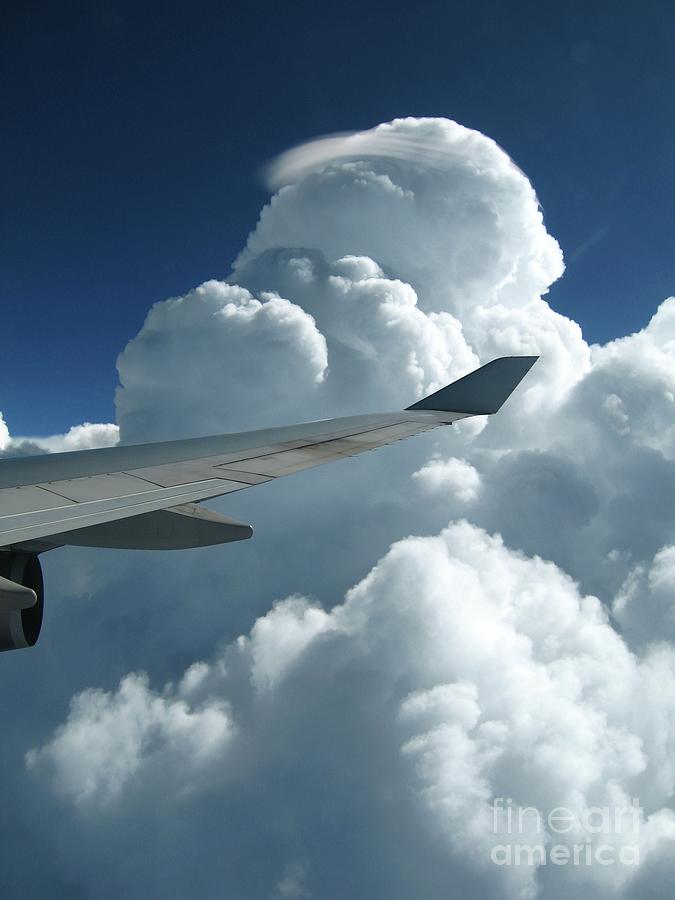The photograph captures the right wing of an airplane during flight on a sunny day, taken from a window seat. Dominating the scene are vast, fluffy cumulus clouds that cover roughly 80% of the image, creating a striking contrast against the deep blue sky that almost turns black towards the top left corner. The airplane wing itself, a sleek gray metal with a slightly curved tip, stretches across the center to the left, where intricate details such as the movable flaps and a dark line indicating their motion can be seen. The engine is partially visible towards the far left side of the wing, slightly obscured but still discernible. The image is marked with a "Fine Art America" watermark at the very bottom right, adding a subtle touch of branding to this serene aerial view.